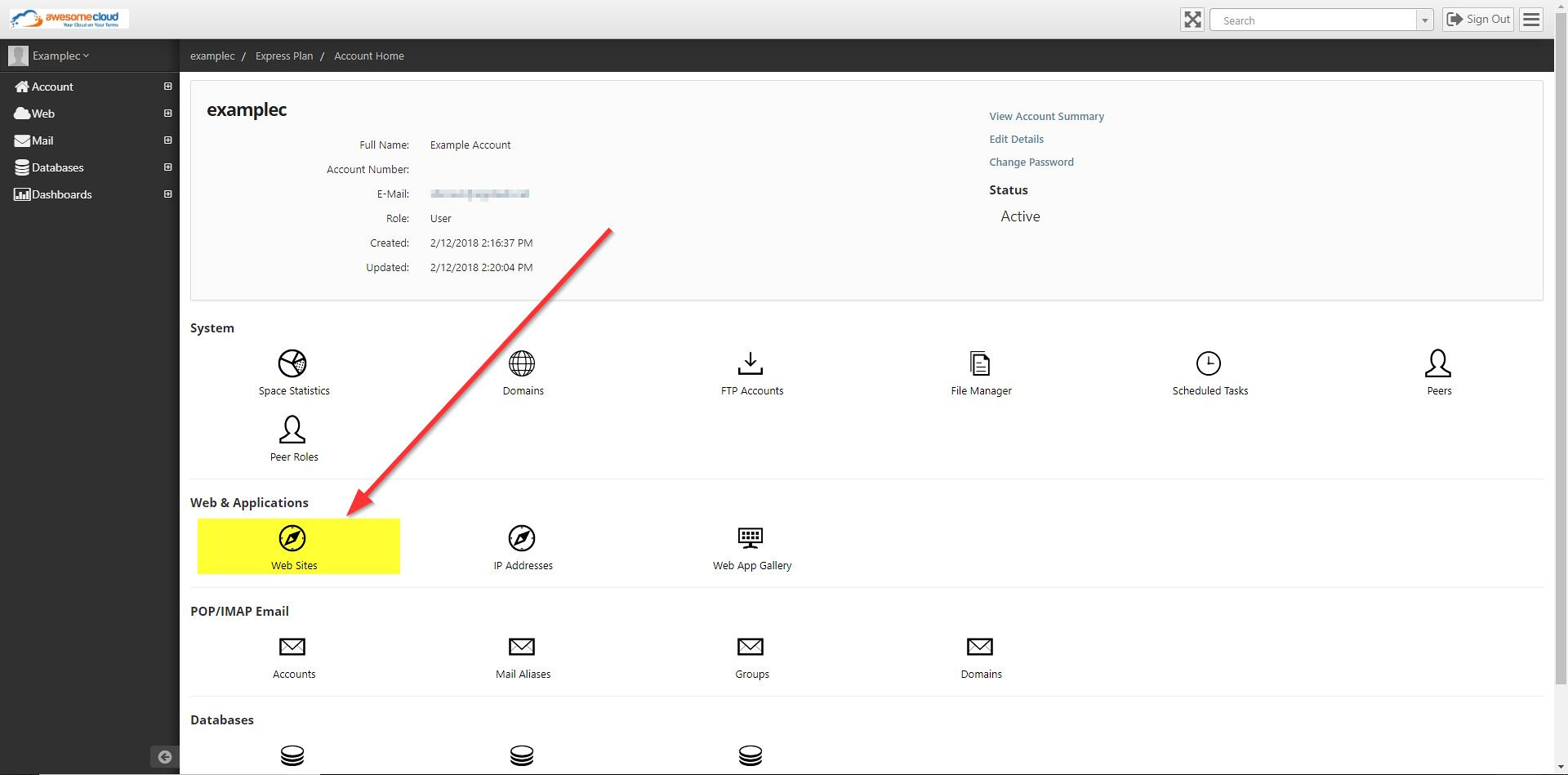This screenshot displays the user interface of "Awesome Cloud," a cloud or internet management platform, offering a comprehensive set of tools and features. The layout is predominantly white, with a sleek dark gray sidebar for navigation on the left side. 

In the top-left corner, there is a distinctive icon along with the text and logo "Awesome Cloud," indicating the branding and ownership of the software. The sidebar is populated with menu items for key sections: Account, Web, Mail, Databases, and Dashboards, enabling swift access to different functionalities.

The main body of the page, characterized by a white background, features a structured grid of icons divided into several labeled sections. 

1. **System:**
   - **Space Statistics**
   - **Domains**
   - **FTP Accounts**
   - **File Manager**
   - **Scheduled Tasks**
   - **Peers**
   - **Peer Roles**

2. **Web and Applications:**
   - **Websites** (highlighted in yellow with a prominent red arrow, indicating the focal point of this screenshot or a specific instruction)
   - **IP Addresses**
   - **Web App Gallery**

3. **POP/IMAP Email:**
   - **Accounts**
   - **Mail Aliases**
   - **Groups**
   - **Domains**

4. **Databases** (separated by a line or a visible break at the bottom).

Each section is clearly defined and organized, making it easy for the user to navigate and manage their resources effectively. The highlighted "Websites" icon with the accompanying red arrow suggests an instructional component or a guided tour within the software interface, directing the user's attention to this particular feature.